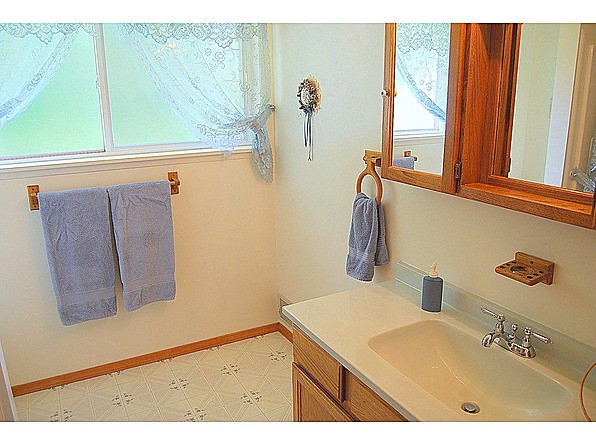The image depicts a cozy bathroom with tastefully chosen decor. A window, adorned with sheer white curtains featuring a delicate light blue doily design along the top, allows natural light to gently filter in. The walls are painted a rich cream color, creating a warm and inviting ambiance that seamlessly extends to the vinyl floor, which is patterned with a square design and light gray accents. A wooden towel bar, situated on the wall, holds two neatly hung bath towels. The focal point of the room is a single bowl sink, set in a dark wood cabinet, providing a striking contrast to the lighter tones. Above the sink, a wooden framed mirror with two flaps—currently open—adds a rustic charm to the functional space.